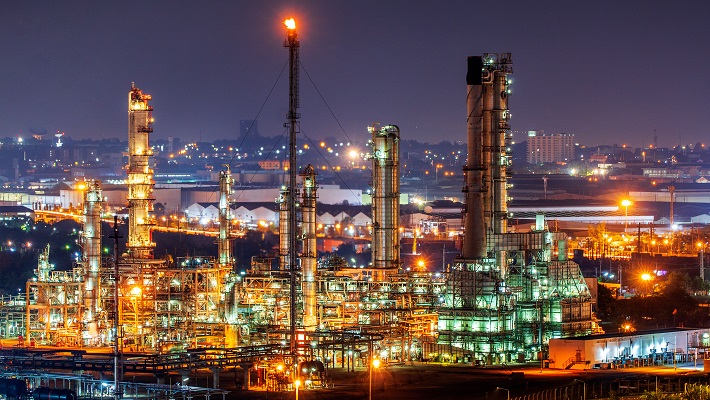This AI-generated image depicts a nighttime cityscape of a populous, industrial area, primarily showcasing an oil refinery. The artistic style eschews realistic textures in favor of a cubist approach. The foreground is dominated by a brightly lit strip of buildings adorned with several smokestacks and towers. Central to the image is an elongated smokestack featuring a prominent, glowing red bulb at the top. The area is bathed in amber and orange lighting, contrasted by the glow from the interior of a green building on the right. The background reveals a slightly lighter, magenta-tinged skyline under a magenta sky, with scattered lights and visible structures like a hotel and other high-rise buildings. Additionally, there’s a river and a bridge visible in the distance. The overall high-quality image is detailed, capturing numerous scaffolds, tubes, and maintenance sheds arranged around the compound, essential for refinery operations. One of the tallest towers features a visible flame, likely for burning off petroleum byproducts.